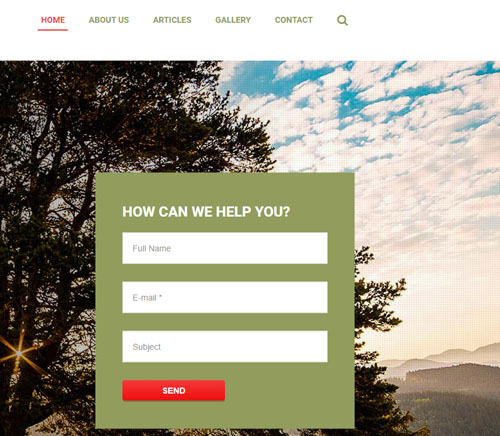The image depicts a serene landscape featuring a backdrop of lush green trees under a brilliant blue sky dotted with numerous clouds. Sunlight filters through the foliage, casting a radiant glow across the scenery. Superimposed onto this natural canvas is a green rectangular section containing the text "How can we help you?" along with fields labeled "Full Name," "Email" (marked with an asterisk), and "Subject." Additionally, a red rectangular section includes text in both sand and white colors. The navigation bar of the webpage is visible, where "Home" is highlighted in red, "About Us" is in gray, and other menu options like "Articles," "Gallery," and "Contact" are also displayed in gray. A magnifying glass icon signifies the search functionality.